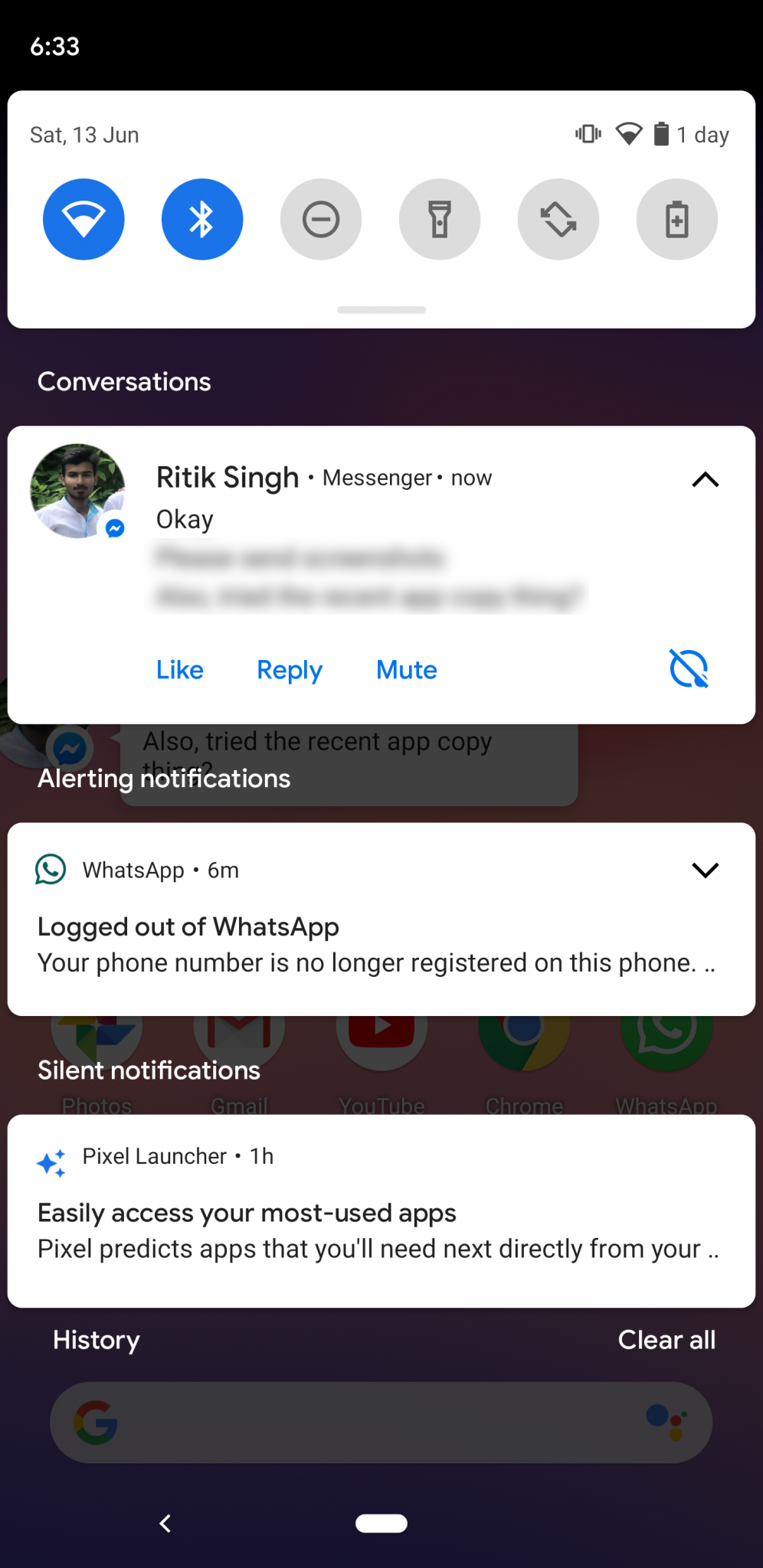The image is a vertically-oriented rectangular interface with a black background. In the upper left corner, the number "633" is displayed in white. The interface is divided into several sections, each containing white rectangles arranged horizontally.

1. **Top Section**: 
   - **SAT 13 June**: This is the date displayed.
   - **Battery and Connectivity Icons**: Depicts various icons indicating battery and connectivity status, including Wi-Fi bars and a battery icon, both indicating "one day." There are also different status icons: two blue circles (representing data/Wi-Fi and Bluetooth), and four gray ones (Do Not Disturb, Flashlight, Screen Rotation, and Battery Saver).

2. **Conversations Section**:
   - **Header**: The word "Conversations" is written in white.
   - **Subheader**: Contains a contact name, "Ritik Singh," labeled under "Messenger Now." Following this are the options "Like," "Reply," and "Mute" in blue text. Part of the message is blurred out, with only "okay" legible.

3. **Notification Bar (Bottom Right)**:
   - Contains a blue circular icon with a diagonal line, implying an option to fold up the notification. Next to it, an upward arrow symbolizes the functionality to expand or collapse notifications.

4. **Alerting Notifications**:
   - A segment labeled "Alerting notifications" appears, followed by another white rectangle detailing a WhatsApp message received "six minutes ago." The message states, "Logged out of WhatsApp. Your phone number is no longer registered on this phone…" with text trailing off.

5. **Silent Notifications**:
   - This section is marked "Silent notifications" in white on a black background.

All sections and text are delineated clearly, emphasizing essential information such as connectivity status, ongoing conversations, and recent notifications in a structured layout.